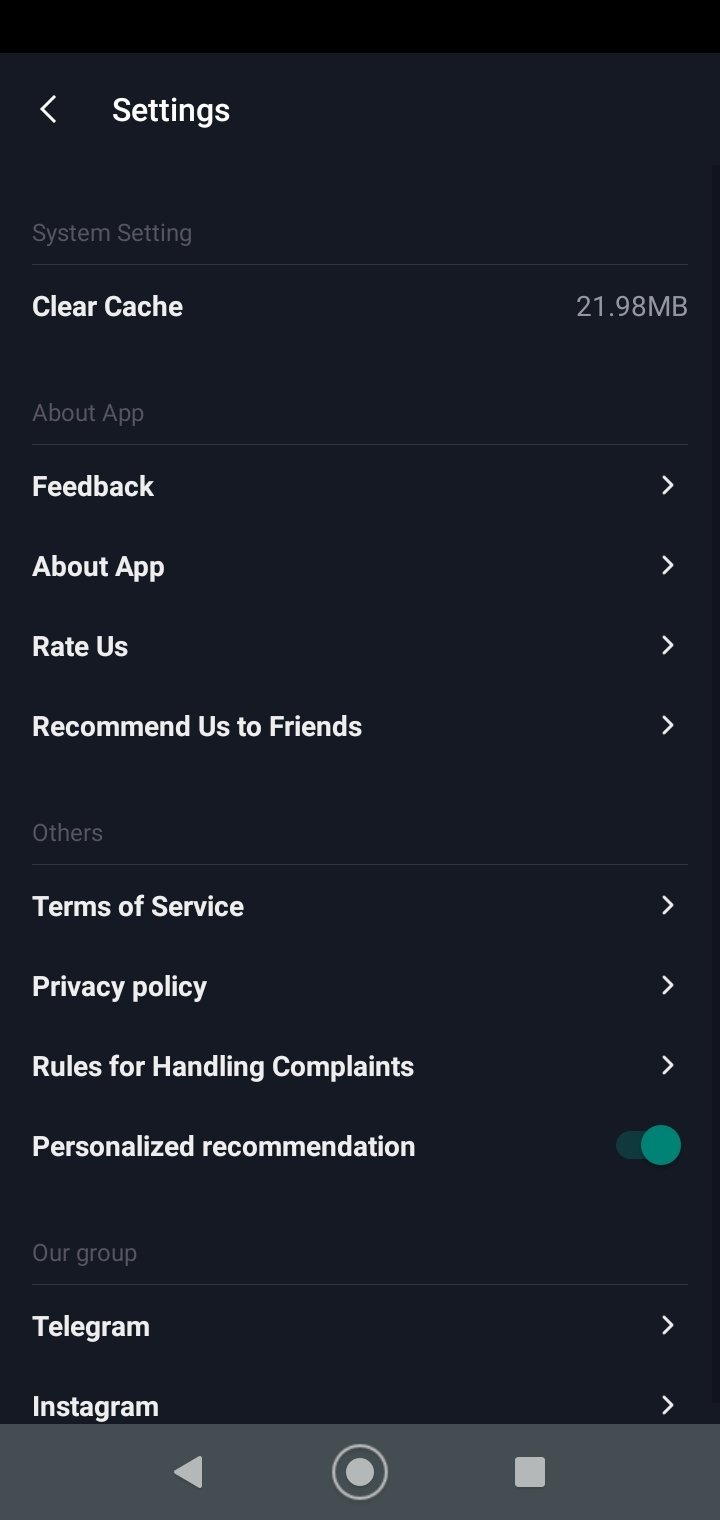The image showcases a phone displaying a settings menu with a black background and white text. At the top, there is a left-facing arrow, indicating a back navigation option. Below this, there's a section titled "System Settings," highlighting a "Clear Cache" option with a cache size of 21.98 MB. Following this, several other options are listed: "About App," "Rate Us," and "Recommend Us to Friends."

Further down, there is a section titled "Offers," which includes links to "Terms of Service," "Privacy Policy," "Rules for Handling Complaints," and "Personalized Recommendations." Notably, the "Personalized Recommendations" option is marked with a green solid circle, distinguishing it from the other options. 

At the bottom of the menu, under the section labeled "Our Group," there are links to Telegram and Instagram, both accompanied by right-facing arrows. 

The image's only icons are those standard on a phone's bottom navigation bar: a left arrow for back navigation, a solid white circle in the center, and a white square representing the home button.